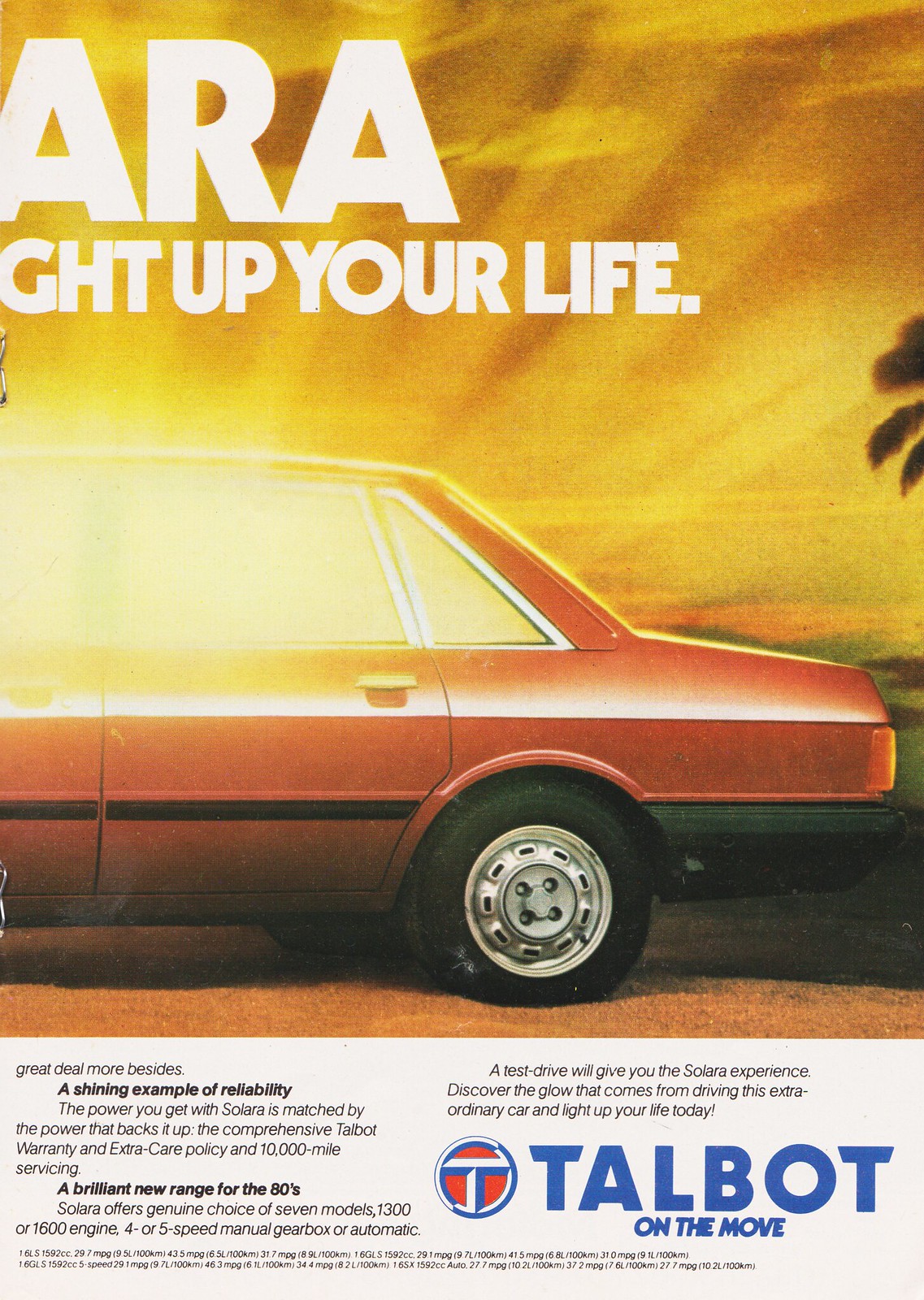This vintage car advertisement showcases an older model with a vibrant sunshine-themed backdrop. The upper section of the ad features a bright sunshine gold background, complete with radiant sun rays, creating an illuminating effect. Prominently placed in large, white letters are parts of the phrase "ARA... GHT up your life," where "ARA" is significantly larger. The focus of the image is on the rear half of an orange car, bathed in sunlight that gleams off the side windows and highlights the vehicle's reddish-orange paint. Visible details include the brightly lit rear window, the black rubber on the rear bumper, and the distinctive orange-red taillights with a touch of yellow. The bottom portion of the ad contains several lines of text boasting the car's reliability and 10,000-mile servicing policy, phrases like "A shining example of reliability," and "A brilliant new range for the 80s" stand out. On the lower right, in blue lettering, it reads "Talbot on the move" accompanied by the Talbot logo.